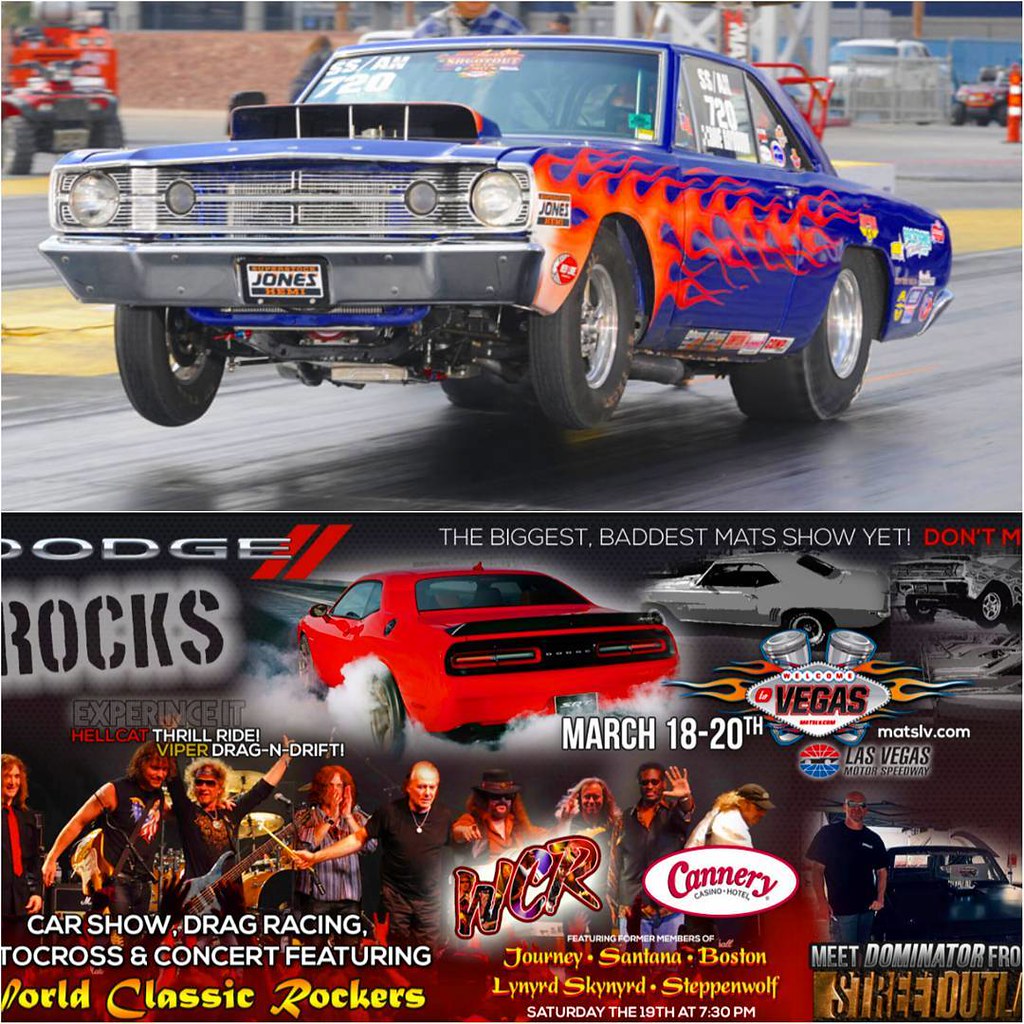This poster is an advertisement for a car show event taking place from March 18-20 at the Las Vegas Motor Speedway, featuring a range of activities including a car show, drag racing, motocross, and a concert. The poster is divided into two sections:

The top section showcases an antique blue car, named Ritz-Jones, with its hood raised and front wheels off the ground, as if launching from a drag race. The car appears on a wet road set against a backdrop of a short brown wall. Notably, the blue car has orange flames on the sides, a hood scoop, and various decals on its windshield and side windows.

In the bottom section, there is a detailed promotional flyer. It highlights the slogan "The biggest, baddest Mats show yet!" alongside the event dates and the venue, with the logo of the Las Vegas Motor Speedway prominently featured. The text is colorful, straddling hues of gray, yellow, red, and white. "Dodge Rocks" is displayed on the left side, pointing to Dodge's sponsorship of the event. The event will include thrilling experiences with high-powered Dodge vehicles such as the Hellcat and Viper, as well as drift demonstrations.

The bottom picture within this section shows the back of a red car with details around it including an announcement of the concert featuring world-class rockers: former members of Journey, Santana, Boston, Lynyrd Skynyrd, and Steppenwolf, performing on Saturday the 19th at 7:30 pm. The right section of the flyer also indicates the chance to meet "Dominator" from Street Outlaws, though parts of this information are incomplete. The poster effectively combines vibrant images and key details to attract attendees to this multifaceted automotive event.